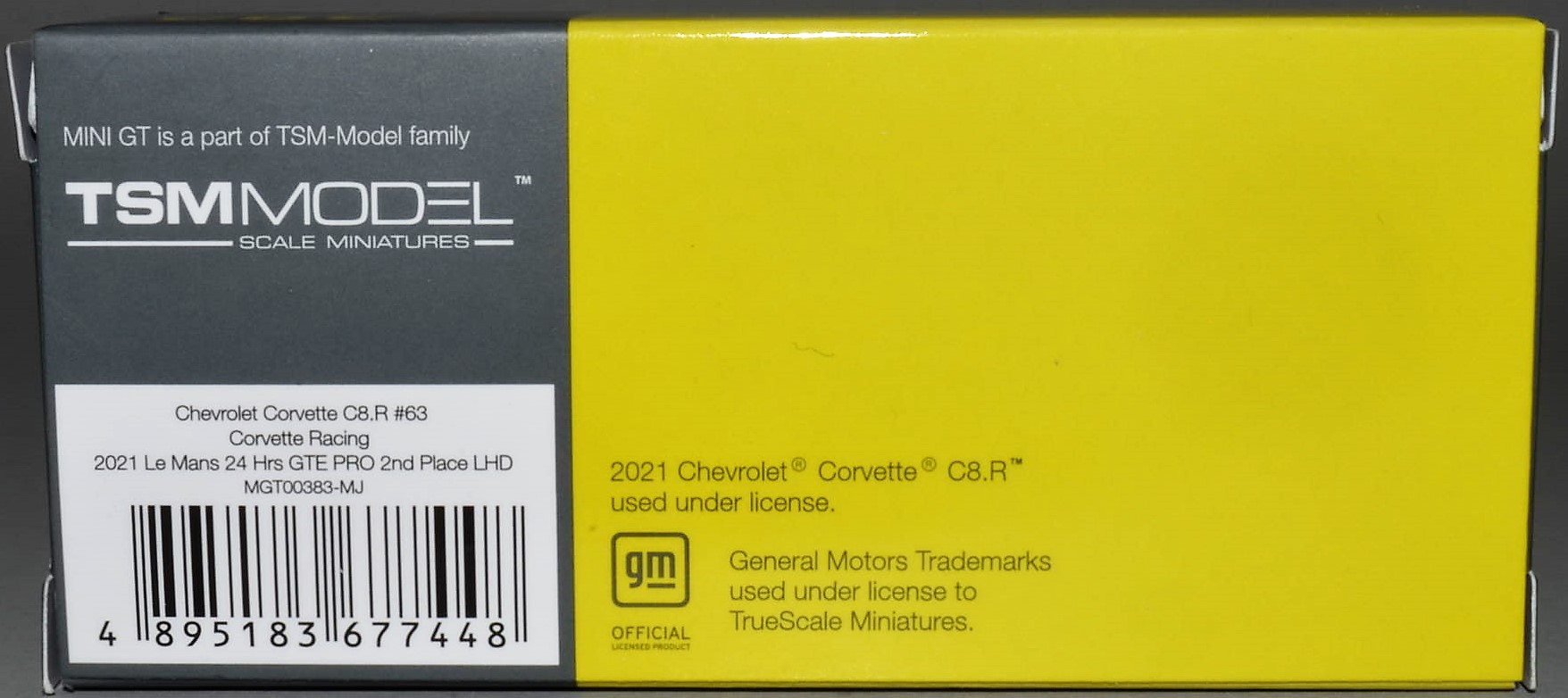This close-up image features the back of a rectangular box, showcasing a detailed miniature model product. The box is divided into two sections: the left third is a dark gray with lighter shades towards the bottom, while the right two-thirds are bright yellow. There’s a clear text demarcation between these sections.

On the yellow portion, black text reads, "2021 Chevrolet Corvette C8.R," followed by a copyright notice, "© Chevrolet," and a trademark declaration, "C8.R™ used under license." Below this, it states, "Official Licensed Product," and "General Motors trademarks used under license to True Scale Miniatures."

The gray portion contains white text, featuring the Mini GT logo with the statement, "Mini GT is part of the TSM Model family," followed by, "TSM model scale miniatures." Below this, a black-and-white striped UPC barcode with the number "4895183677448" is present. Above the barcode, it reads in black text, "Chevrolet Corvette C8.R #63 Corvette Racing 2021 Le Mans 24 Hours GTE Pro Second Place LHD MGT 003833-MJ."

This box is for a highly detailed model car, emphasizing its authenticity and alignment with licensed products from General Motors.